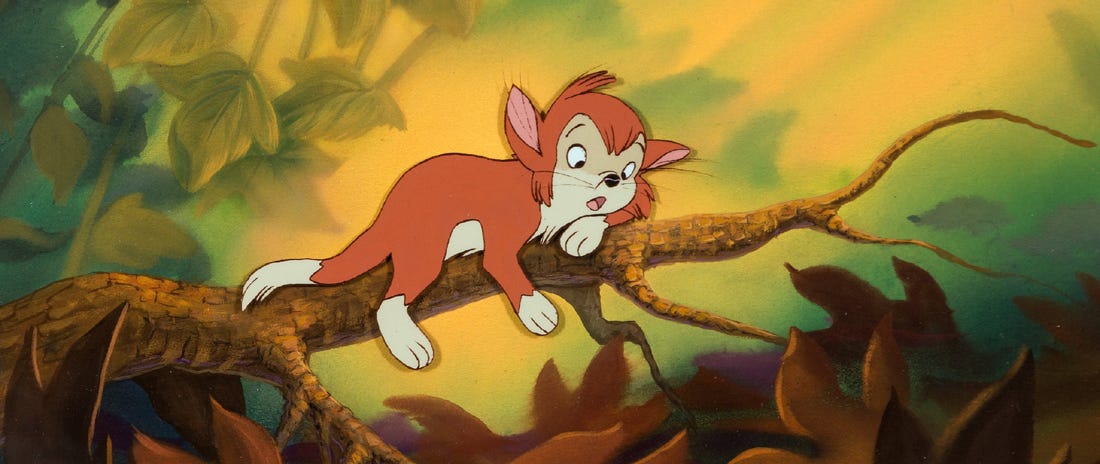This is a detailed computer-generated color illustration, likely inspired by a Disney production, showcasing a cartoon character. The image is in a wide, horizontal, landscape format, centered around a large, horizontal tree branch that runs from the bottom left to the top right. The focal point is a wild animal, possibly a lion or a monkey, but notably reminiscent of the cat from "Tom and Jerry." This cartoon creature is illustrated with a brown, brick-colored coat, a cream-colored belly, and a beige face. It has white paws and the tip of its tail is also white. Its ears are pink inside. 

The animal is stretched out on its stomach on the tree limb, with one paw under its head and the others dangling down. Its eyes are wide with a surprised expression, and its brows are raised. The character is looking down towards a cluster of gold leaves on the ground below, with its mouth open in surprise. The background features out-of-focus leaves and plant life in shades of gold and green, illuminated by a soft yellow light, creating an ambient jungle setting.